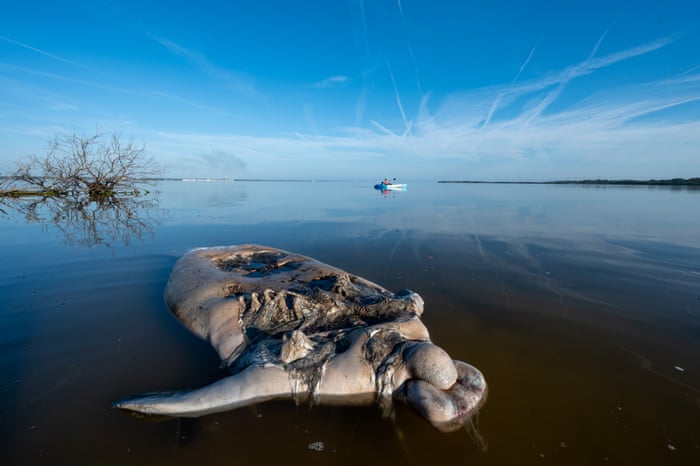The image depicts an open expanse of still water, likely a lake, with a distant shoreline stretching from left to right near the horizon. On the left, just below the shoreline, a small landmass with some trees or bushes juts out. The rock formation central to the image is light gray with darker gray patches, uniquely shaped with protrusions and indentations. It rises from the bottom right of the image, curving upward and to the left. Detailed lines and markings cover its surface, with a particularly noticeable thin piece jutting out to the left. In the bottom center of the image, a faint number is visible.

In the foreground, a decaying mass that looks like a dead animal or fish floats in the water, colored pink and gray, with a disintegrating, fleshy texture. This mass dominates the lower portion of the image, appearing quite grotesque. 

Further in the background, a small, white boat with blue sides drifts in the distance, possibly carrying a couple of people. The water is clear, reflecting the surrounding elements, including a dead tree on the left whose reflection is visible. The sky above is blue, dotted with a few clouds and streaks of plane smoke. The overall scene is serene yet marred by the presence of the decaying mass in the foreground.